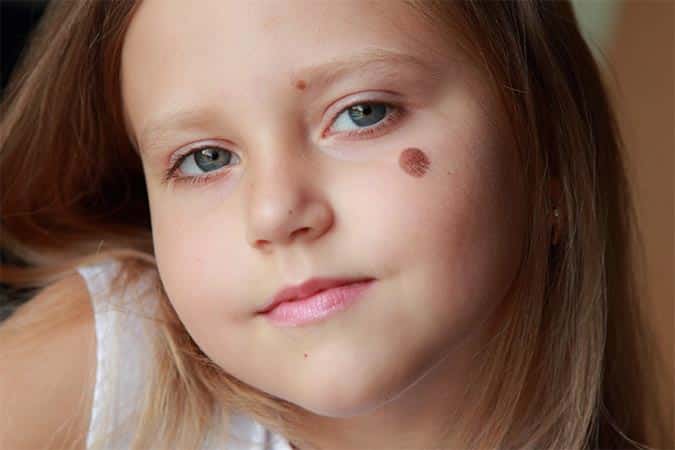This image is a close-up photograph of a sweet-looking young girl with expressive blue-green eyes and light brown hair that almost appears blonde. She's gazing directly into the camera, showcasing her round face adorned with two moles: one situated at the edge of her left eyebrow near her nose and another under her left eye, on her cheek. Her light brown hair cascades down, partially covering what seems to be a white, sleeveless top or undershirt, revealing just the top of her shoulder and a glimpse of an ear that might be adorned with an earring. Additionally, the child is wearing light pink lipstick, giving a touch of color to her lips. The photograph, taken during the daytime, brings out the delicate features of her face in vivid detail.